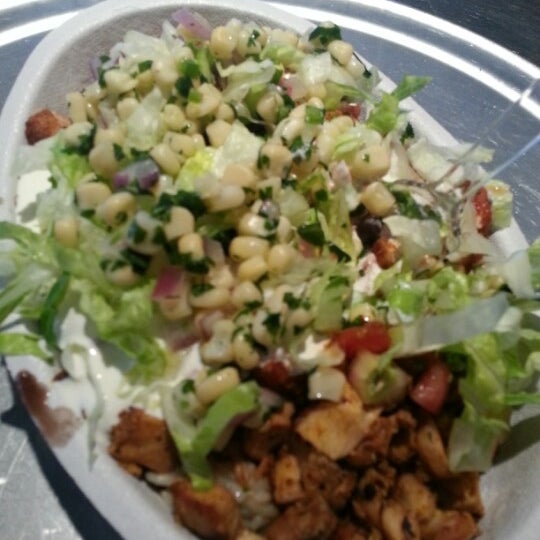This close-up photograph captures a to-go salad placed in a white paper bowl, set atop a silver tray or table. Central to the image, the salad features a bed of green lettuce, yellow corn possibly garnished with cilantro, diced onions, cream-colored beans, and scattered red tomatoes. In the bottom corner of the bowl, there is brown, grilled chicken seasoned to perfection. A clear plastic spoon is prominently inserted into the salad, adding to the takeaway appeal. A white sauce, likely sour cream, is visible on the side, enhancing the dish's rich visual texture. The entire setup rests on a gray-colored surface, emphasizing the fresh and vibrant appearance of the food.